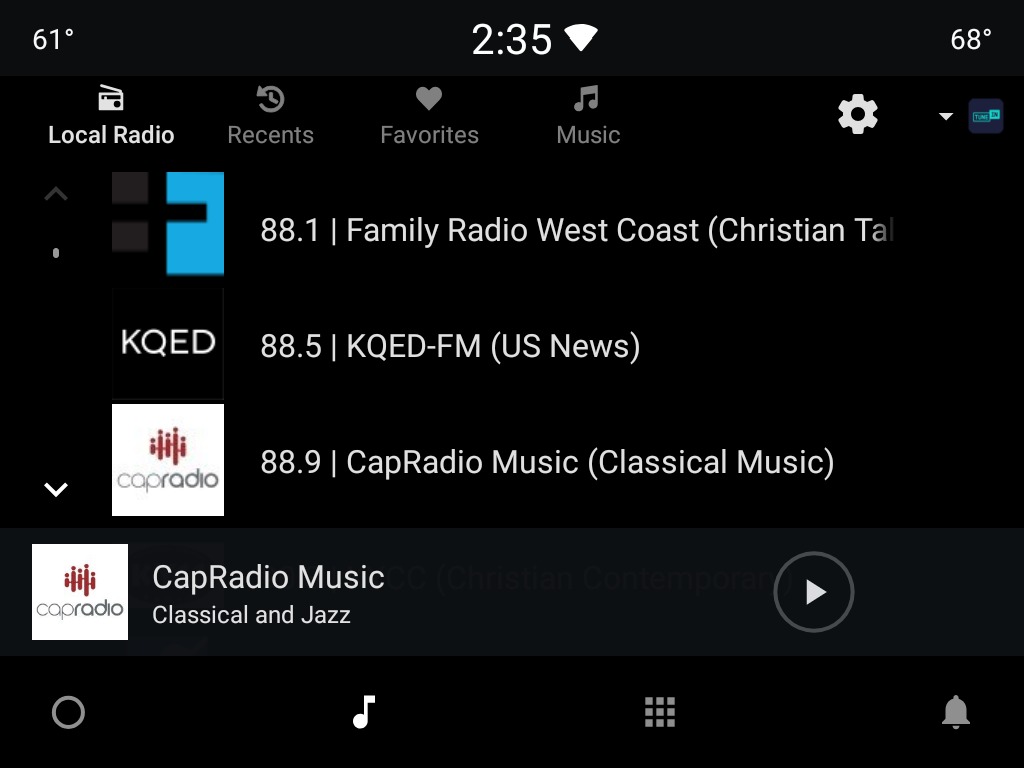The image is a screenshot from a device displaying a local radio interface. The background is predominantly black, creating a high-contrast view for easy readability. At the top left corner, the current temperature is shown as 61 degrees, while the top right corner displays a different location's temperature at 68 degrees. The time is indicated as 2:35, accompanied by a Wi-Fi signal icon. 

Several navigation options are visible, including "Local Radio," "Recents," "Favorites," and "Music." There's also a gear icon presumably for settings. As you move down the interface, there are up and down arrows on the left side for scrolling through the stations. 

The currently selected station is "88.1 Family Radio, West Coast, Christian Taw," although it appears to be truncated. Below this, "KQED-FM" is listed, labeled as "U.S. News" on the 88.5 frequency. Further down, "88.9 CAP Radio Music" is noted, with a description highlighting "Classified Classical Music."